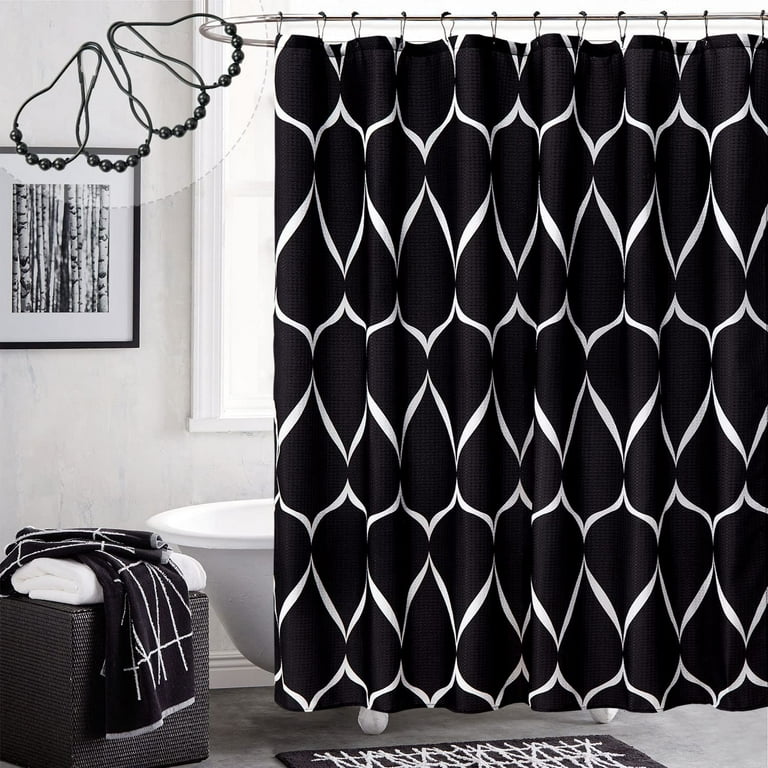This photograph showcases a modern, well-kept bathroom with a sleek black-and-white theme. The focal point of the image is the black shower curtain adorned with intricate white lines forming repeated shapes, which is pulled mostly closed. Behind it, the traditional white bathtub, elevated on feet, peeks out from the left side and is partially obscured by the curtain. The walls of the bathroom are white, enhancing the contrast of the black elements.

In the space to the left of the tub, a hamper is topped with a neatly folded white towel, and another towel or a piece of the shower curtain with a matching black-and-white pattern drapes over the side. A matching bath mat with a similar black and white design lies on the gray floor in front of the tub.

Adding to the decor, a framed black-and-white photograph depicting a close-up of trees is positioned above the bathtub. A large window behind the shower curtain allows natural light to filter in, partially obscured by the curtain. Additionally, the top corner of the image features a semi-transparent circle containing four shower curtain clips, further emphasizing the bathroom's modern, polished aesthetic.